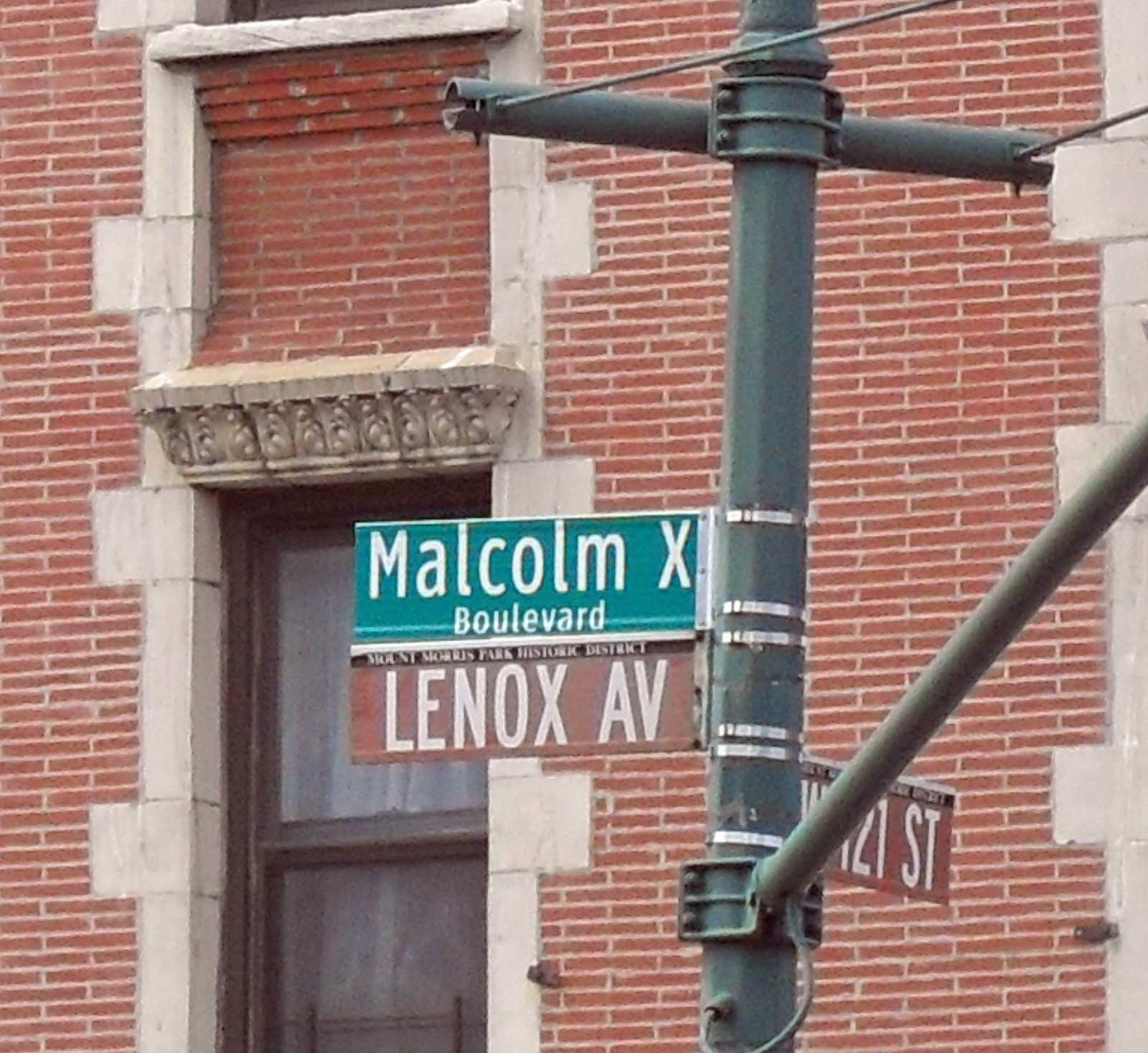In this close-up image, we see a street sign positioned against a backdrop of a brown brick building. The street sign is mounted on a dark green, tall, vertical post, with another angled post attached to its right side. Due to the image's framing, the endpoint of the angled post and any additional signage it might support are not visible. A horizontal bar extends from the top of the post, which has wires emerging from it, disappearing beyond the picture's edge.

The central feature of the signpost is a dark green sign with white lettering that reads "Malcolm X Boulevard." Directly beneath it, a brown sign also in white text declares "Lenox Avenue." On the opposite side of the post, another brown sign is partially visible, and though the text is unclear, it seemingly indicates "West 21st Street."

Behind the signpost, the brown brick building is notable for its architectural details. One of the windows, framed in dark brown and set in a cement border, has a white curtain drawn across it, adding a touch of domesticity to the urban scene.